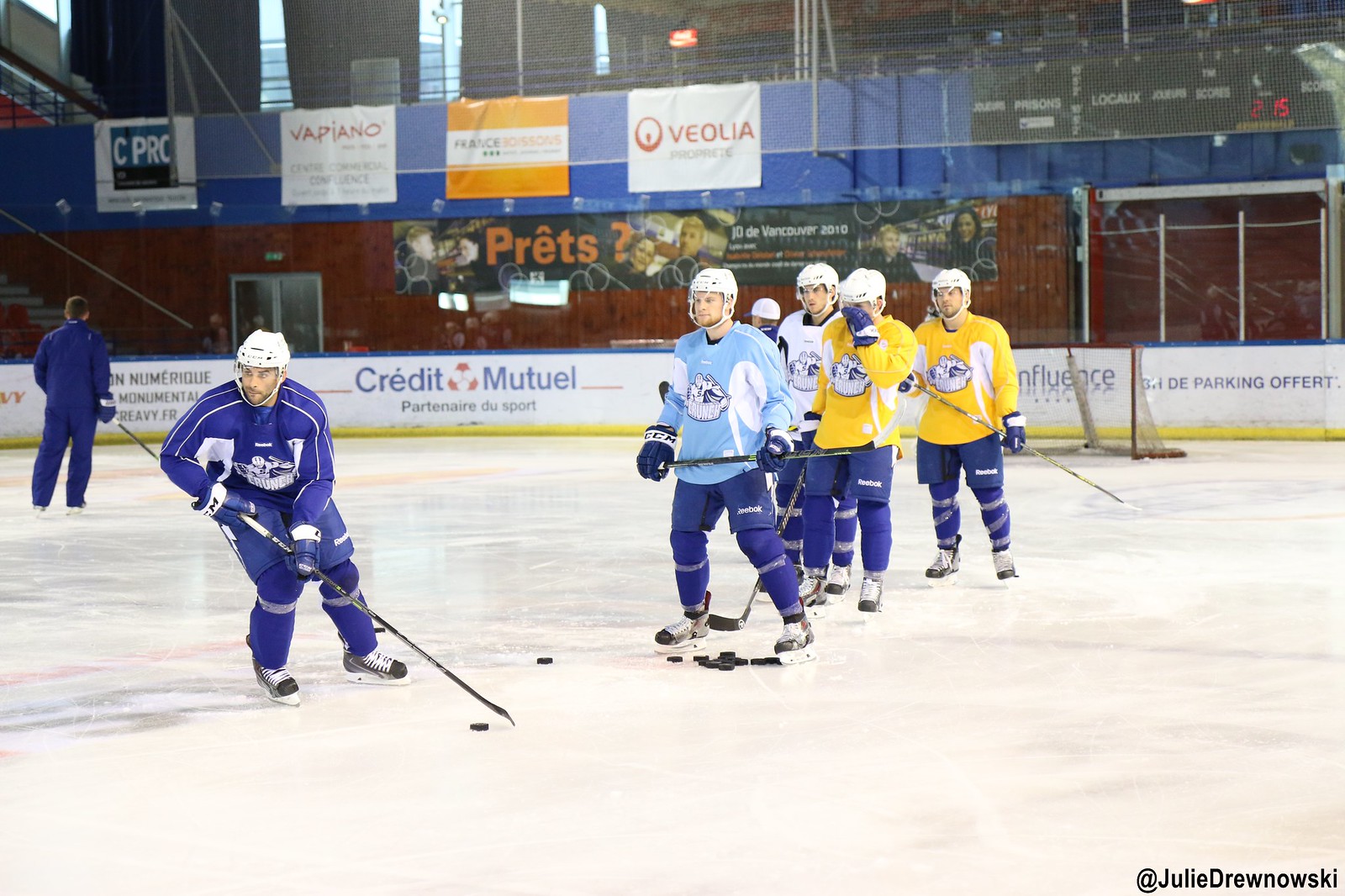The photo captures a hockey team practicing on the ice rink, possibly in a shootout drill. Around a dozen pucks lie in a pile on the ice, with a player in a blue uniform shooting one of them. He is first in a lineup of players, each clad in different colored jerseys but uniformly wearing blue pants and white helmets. Immediately behind the shooter, a player wears a lighter, powder blue jersey, followed by players in yellow and finally one in white. All players share a common insignia on their jerseys, though its details are unclear. Advertisements in French, including "Crédit Mutuel," line the barrier in the background, suggesting the rink might be in Quebec, Canada, or France. Banners above the barrier feature names like Veola, Papiano, and Seapro. A scoreboard on the upper right corner displays "2:15." Behind the players, there’s another goal and stands with empty seats. Far left, a non-player in dark blue, possibly an attendant or coach, stands with his back to the camera. The photograph credits @JulieDrewNowski in the bottom right.